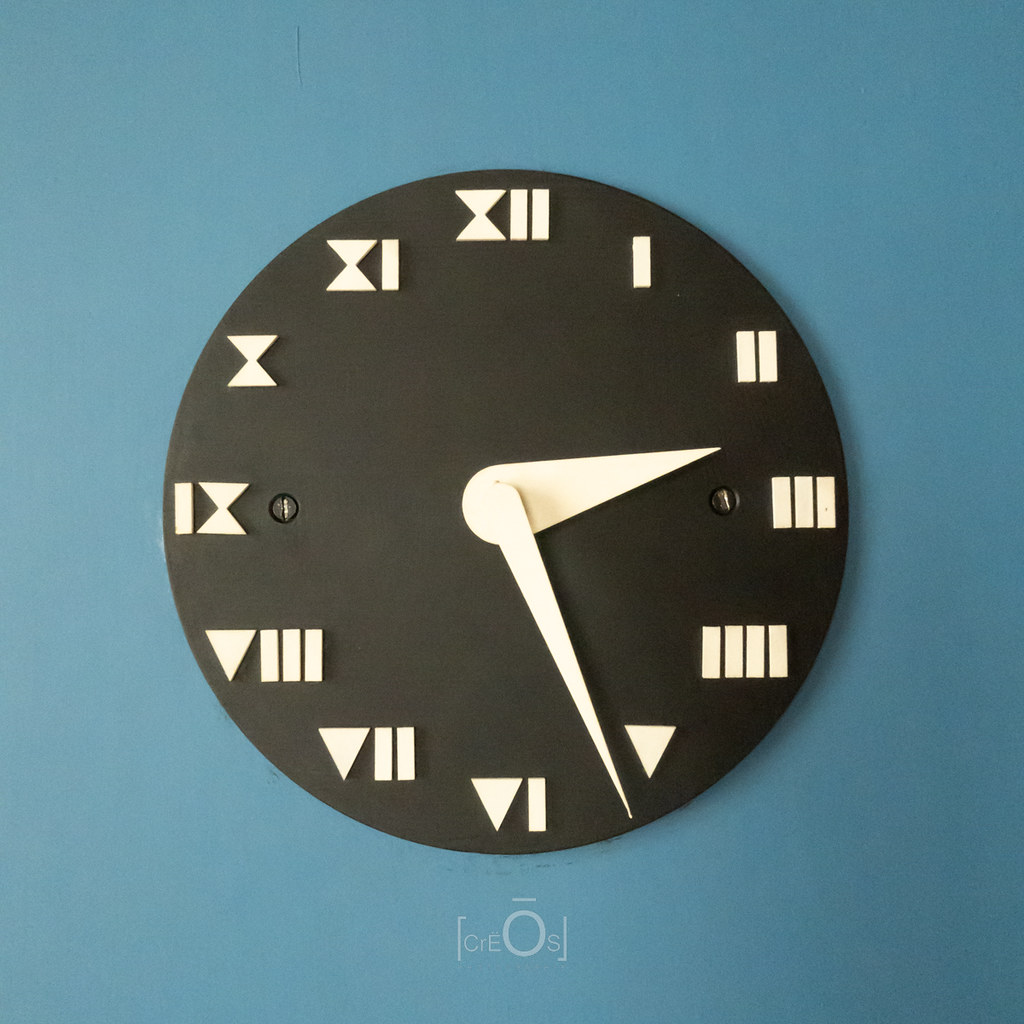In the image, a round, black-faced clock is prominently displayed, bolted securely to a solid, light blue wall. The clock features bold Roman numerals in ivory, but with unique designs where the X resembles an hourglass, and triangles replace the traditional V shape. The thick, short hour hand and the long, slender minute hand, both in ivory, indicate the time as 2:27. Beneath the clock, there's a faded logo with the letters "CRE" followed by a large "O", and then an "S", with lines adorning the start and end of the word and a line above the "O". The photograph, oriented vertically, captures the scene in a well-lit room, emphasizing the striking contrast between the black clock and its blue-green background.